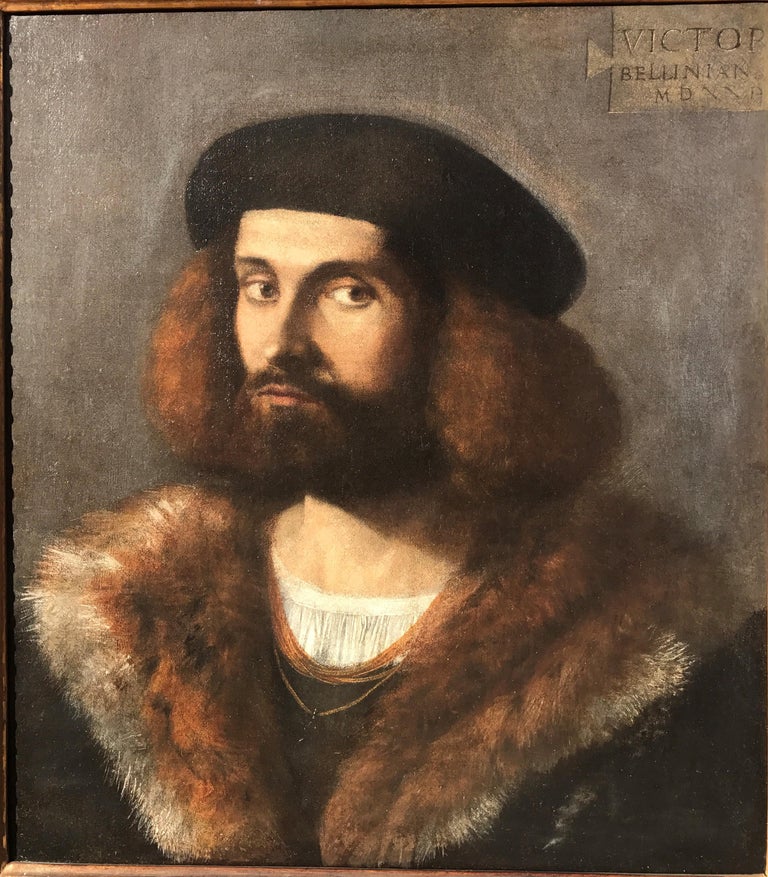This detailed image portrays a Renaissance-era painting of a white man with distinct reddish-brown, long, curly, and frizzy hair that reaches down to his shoulders, meticulously covering both of his ears. He sports a full but not very long beard along with a mustache, and his expressive brown eyes and slightly sideways gaze lend him a contemplative appearance. Adorning his head is a large black beret that holds down his voluminous hair.

The man is clad in layered attire: a white pleated undershirt, topped by a black garment, and finally enveloped in a grand black coat with a light brownish-reddish fur trim that nearly matches the color of his hair. At his neck, he wears a necklace or pendant. 

The painting is framed in a brown-colored frame, set against a gray background that resembles a stone or cemented wall. Intriguingly, in the top right corner, there's an inscription that reads "Victor Bellinon MD NMA" or "Victor Belenian." The overall composition of the portrait, with the man’s sideways glance and the ornate attire, epitomizes the elegance and detail typical of Renaissance portraiture.